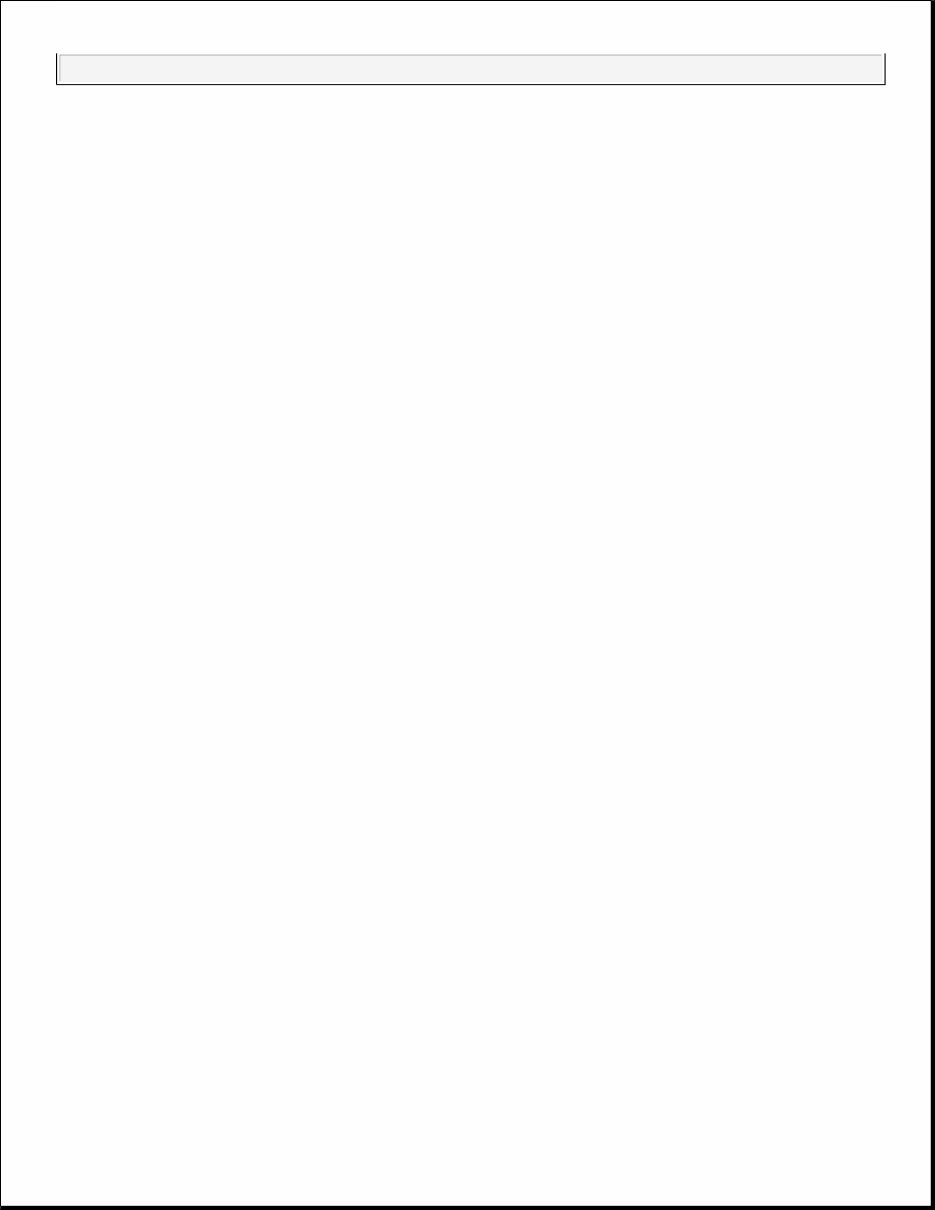Screenshot of a Minimalist Webpage:

This image captures a webpage that is almost entirely devoid of content, showcasing a minimalist and stark design. The background is completely white, creating a clean, uncluttered look. At the top of the page, there is a long rectangular bar that may resemble a search box due to its shape and placement; however, it is outlined in black and appears slightly off-white, with no text or buttons within it, rendering its function ambiguous.

The webpage itself is framed within a tall rectangular area, outlined with a black border. Notably, the borders on the right side and the bottom of the webpage are slightly thicker compared to the left and top borders, adding a subtle variation to the otherwise uniform design. The rest of the page remains entirely blank, featuring no text, images, addresses, or additional elements of any kind, emphasizing the stark and simple aesthetic of the blank webpage.